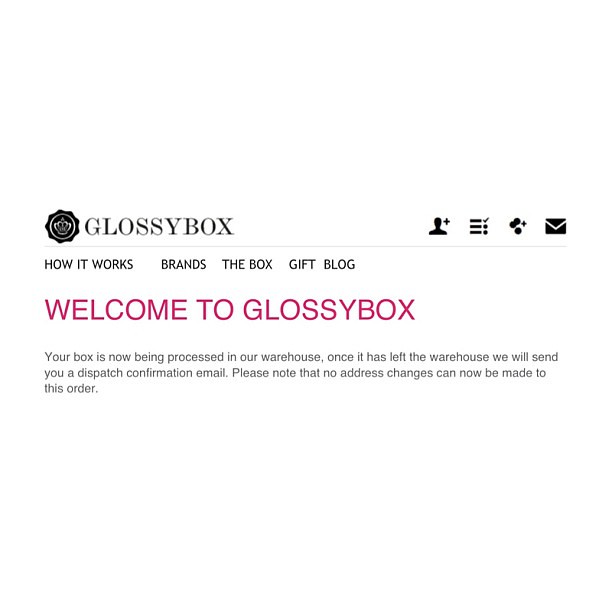The image is a detailed screenshot of the Glossybox website. It features a solid white background with the brand's logo in the top left corner—a black circular emblem with a white circle and a crown inside it. Directly beside the logo, in all caps black letters, it reads "GLOSSYBOX," followed by a light gray horizontal line separating it from the main content. Underneath, a navigation menu lists options in black text: "How It Works," "Brands," "The Box," "Gift," and "Blog." Beneath this menu, large red or pink text warmly greets the visitor with "Welcome to Glossybox." Just below this welcome message, descriptive black text states, “Your box is now being processed in our warehouse. Once it has left the warehouse, we will send you a dispatch confirmation email. Please note that no actual address changes can now be made to this order.” On the top right are four black icons: a profile head with a plus sign, a checklist, an indeterminate icon, and an envelope, with a hamburger menu alongside them, all providing additional navigation options.